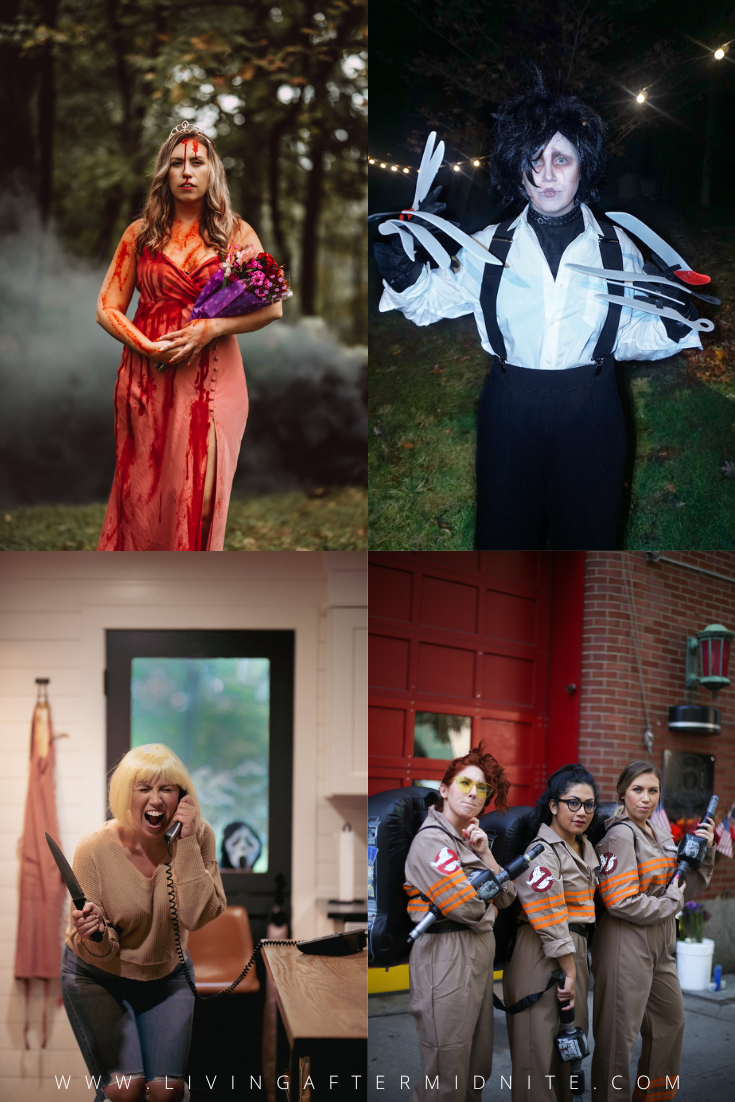The image is a composite of four photographs, each showcasing detailed cosplay by a woman in various iconic horror and fantasy characters. 

In the top left, the woman portrays Carrie from the 1976 film "Carrie," wearing a blood-soaked prom dress, tiara, and holding a bouquet, reminiscent of Sissy Spacek's character. The top right features her as Edward Scissorhands from Tim Burton's 1990 movie, complete with the character's distinct outfit and scissor-like hands. In the lower left, she emulates Drew Barrymore's character, Casey Becker, from the 1996 movie "Scream," dramatically holding a telephone and knife, with the masked Ghostface killer lurking behind her. The lower right photograph includes her alongside two other women, all dressed in Ghostbusters uniforms, standing in front of a large firehouse garage door, evoking the 2016 "Ghostbusters" movie inspired by the 1984 original. 

A website, www.livingaftermidnight.com (note: 'midnight' is spelled 'M-I-D-N-I-T-E'), is faintly visible, possibly attributing credit or providing further context.